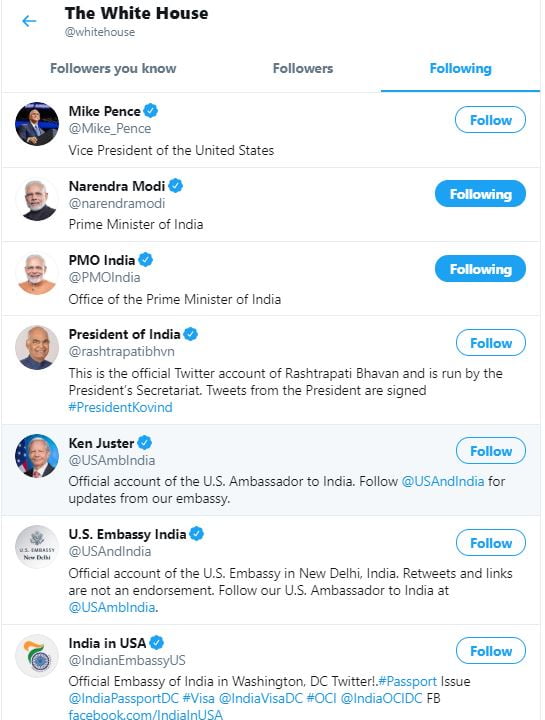The image is a screenshot featuring a list of Twitter accounts with associated follow statuses. The screen shows the following elements:

1. **The White House (@WhiteHouse)** - This account is marked with a blue arrow pointing to the left and the status "Following," which is highlighted in blue, while the other words are in gray.

2. **Mike Pence (@Mike_Pence)** - Displayed as the "Vice President of the United States," with the status indicating "Follow."

3. **Narendra Modi (@narendramodi)** - Listed as the "Prime Minister of India" and marked as "Following," with reference to the official account @PMOIndia.

4. **President of India (@rashtrapatibhvn)** - The account is marked as "Follow."

5. **US Ambassador to India (@USAmbIndia)** - Featured with a follow status of "Follow."

6. **US Embassy India (@USAndIndia)** - Also marked as "Follow."

The background of the image prominently includes the White House.